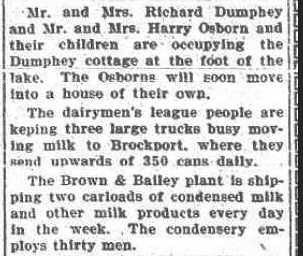The image depicts a newspaper clipping on white paper with black text. It contains three paragraphs of information framed by a very thin gray bar on the left and a thicker black bar on the right, complemented by a thin gray bar and small gray squares. The text reads: "Mr. and Mrs. Richard Dunphy and Mr. and Mrs. Harry Osborne and their children are occupying the Dunphy cottage at the foot of the lake. The Osbornes will soon move into a house of their own. The Dairyman's League people are keeping three large trucks busy moving milk to Brockport, where they send upwards of 350 cans daily. The Brown and Bailey plant is shipping two carloads of condensed milk and other milk products every day in the week. The condensary employs 30 men." The clipping has some small black specks scattered on the white background.